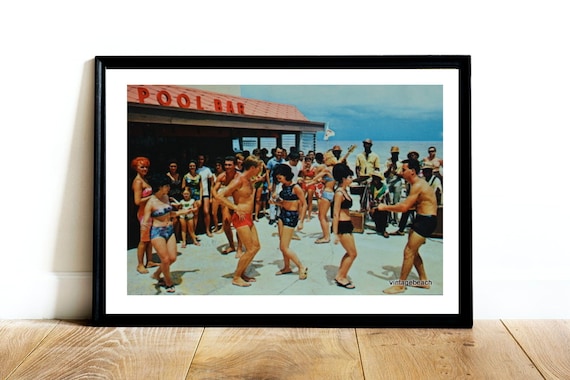The image depicts a black-framed photograph leaning against a white wall on a medium-colored wooden floor. The frame, which casts a light shadow to its left, features a white matting border. At the center of the frame is an aged photograph, possibly from the 1960s to 1980s, showing a lively scene at a beach or poolside bar. On the left side of the photograph, a pink sign with red letters reads "POOL BAR." The scene is bustling with primarily Caucasian men and women in swimwear, dancing on what appears to be a sandy or concrete surface. In the far background, a serene body of water meets the sky on the horizon, and there are four to five dark-skinned musicians visible on the far right, enhancing the joyous atmosphere. The specifics of the hairstyles and conservative bathing suits further suggest the era captured in the photo.